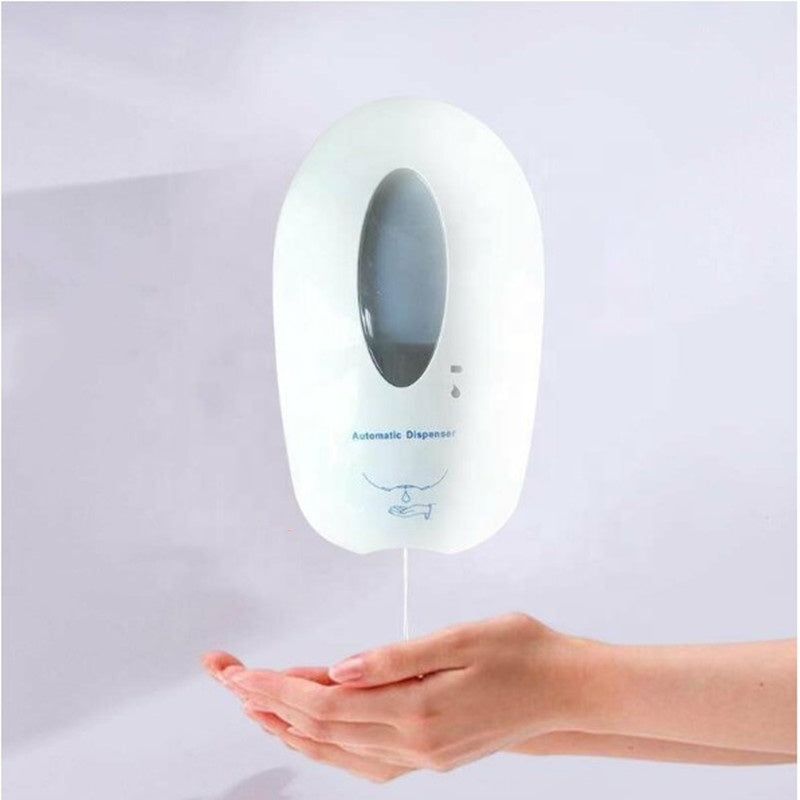This detailed photograph features a pristine, medical stock image of a white, ovular automatic dispenser with blue text that reads "automatic dispenser." The dispenser also displays a small blue diagram at the bottom, illustrating a drop of liquid being dispensed into a hand. The device includes an oval-shaped window showing the remaining amount of cleansing liquid, which is notably low, approximately one-sixth full. The background is a soft, off-white color, creating a clean, clinical setting. Two pale, fair-skinned hands with well-manicured nails are cupped underneath the dispenser, extending from the right edge of the frame to the center. These hands are positioned to catch a thin stream of white liquid soap or hand sanitizer being dispensed.